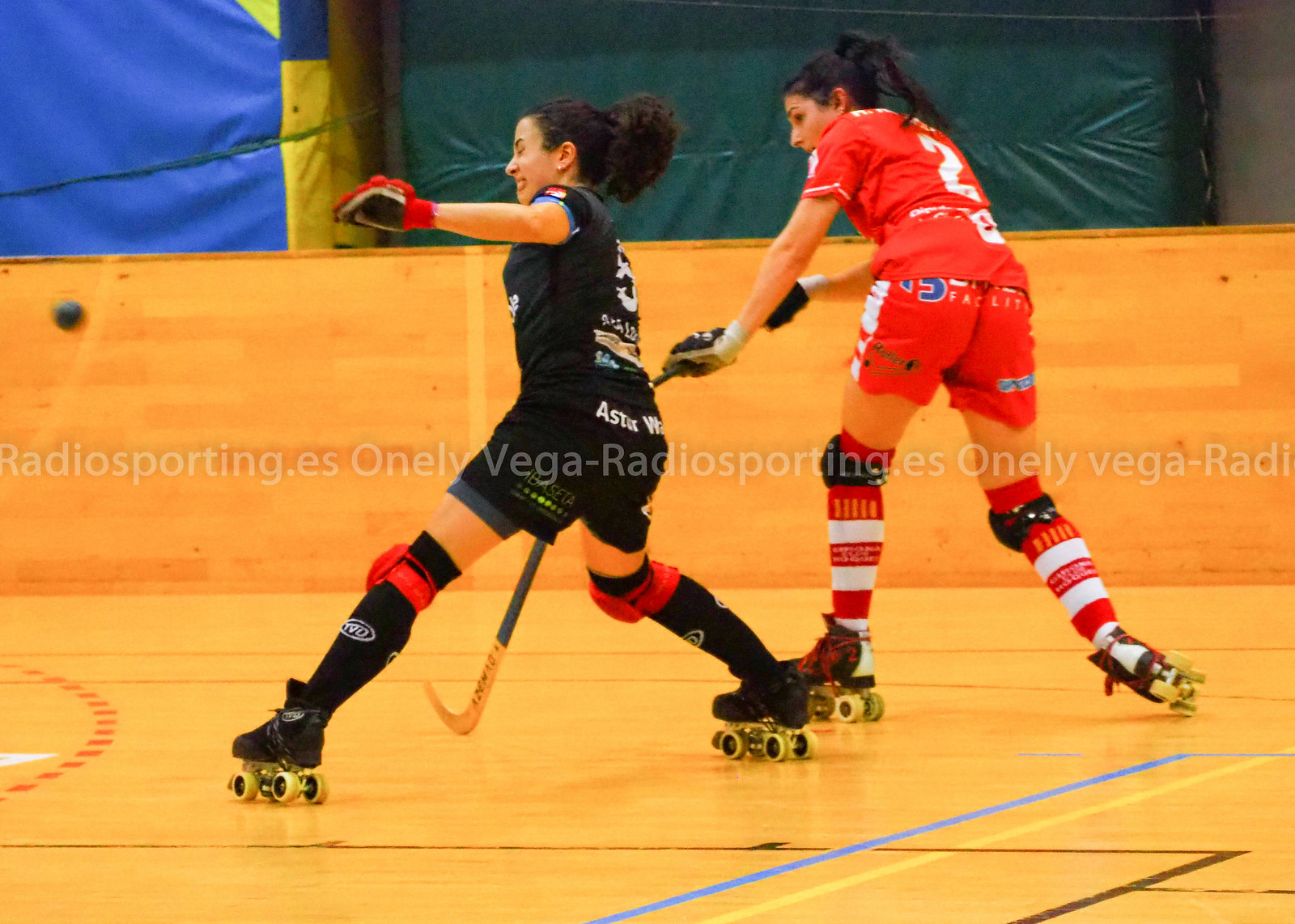The image captures an intense moment during an indoor roller hockey session, set in a gymnasium with a hardwood court. The court features a variety of lines in black, yellow, blue, and dotted red, bordered by a wooden wall and padded areas in green, blue, and yellow. Two women, both with dark hair pulled back, are the focal point, dressed in full roller hockey gear including knee pads, gloves, roller skates with yellow wheels, and holding hockey sticks. On the left side, one woman is clad in a black outfit—black jersey, shorts, socks, and skates, with orange knee pads and matching gloves. Her opponent, positioned slightly behind, is wearing a striking red jersey with white details, red shorts, red socks, and black skates with red laces. Both women are converging toward a black ball suspended in midair, embodying the competitive spirit of the game.